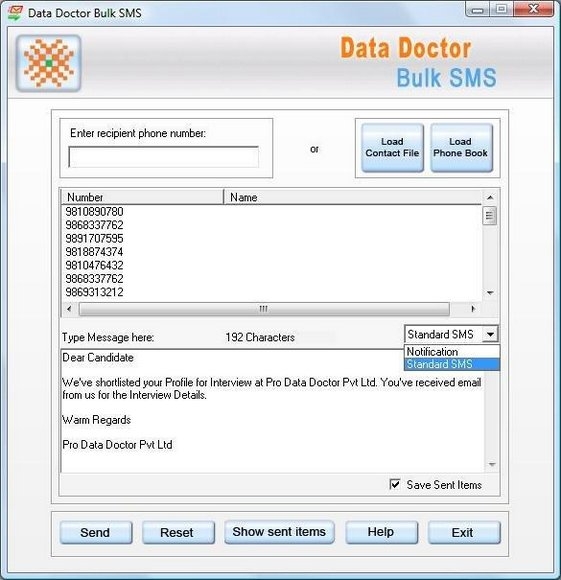Sure! Here’s a cleaned-up, detailed caption for the image description provided:

---

The image shows a computer application window titled "Data Doctor Bulk SMS." At the top right corner of the window, there are minimize, maximize, and exit buttons. Below the title, "Data Doctor Bulk SMS" is repeated, followed by a section labeled "Enter Recipient Phone Number," which includes a text box for manual input. To the right of this text box are two buttons: "Load Contact File" and "Load Phone Book."

Below this section, there's a scrolling menu displaying a list of phone numbers, all starting with the number 9 in the area code. Beneath the scrolling list, there's a label "Type Message Here, 192 characters," accompanied by a dropdown menu offering options to choose either "Standard SMS" or "Notification." Following the dropdown menu is another text box containing a pre-written message: “Dear Candidate, we’ve shortlisted your profile for an interview at ProDataDoctorPVT LTD. You’ve received an email from us with the interview details. Warm regards, ProDataDoctorPVT LTD.”

At the bottom of the application window, there is a row of buttons with various options: "Send," "Reset," "Show Sent Items," "Help," and "Exit."

---